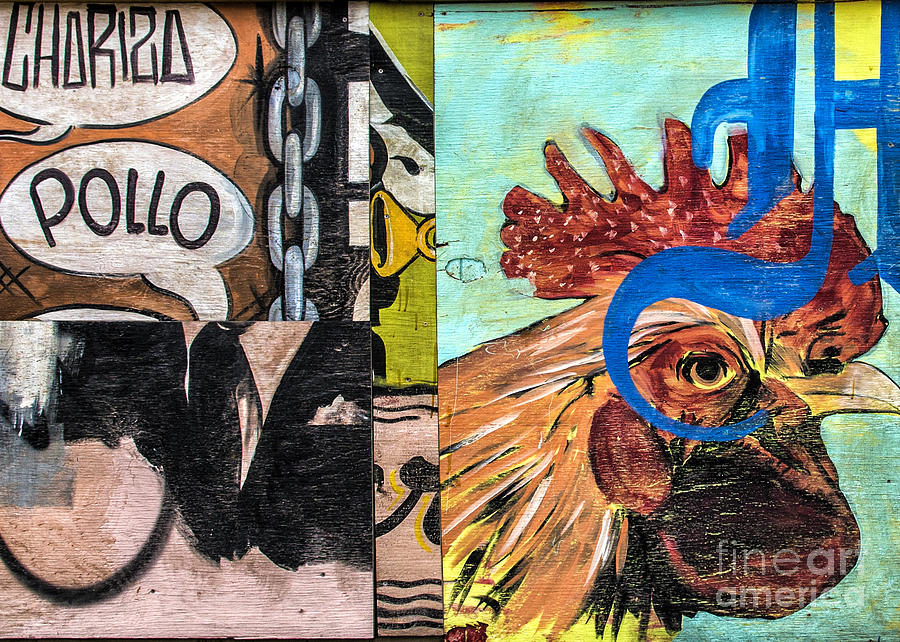The image is a vibrant and eclectic art piece painted and collaged on plywood. Dominating the right side of the collage is a vividly painted rooster, featuring a striking red crest and a plumage in shades of bright reds, oranges, and yellows. The background here is turquoise, adding to the overall vibrancy. To the left, the artwork transitions into a comic-style segment with speech bubbles containing text such as "Teresa," "Pallo," and possibly "Chorizo Pollo." This section also includes a horizontal chain and some form of pipe, possibly colored blue. The central strip dividing the two main sections is narrower and composed of abstract colors. In the bottom left corner, there is what seems like an up-close view of graffiti, partly obscured, possibly depicting a cut-off name. The image is marked by its dynamic use of bold, bright colors, creating a captivating, street-art-inspired collage that invites lengthy contemplation.